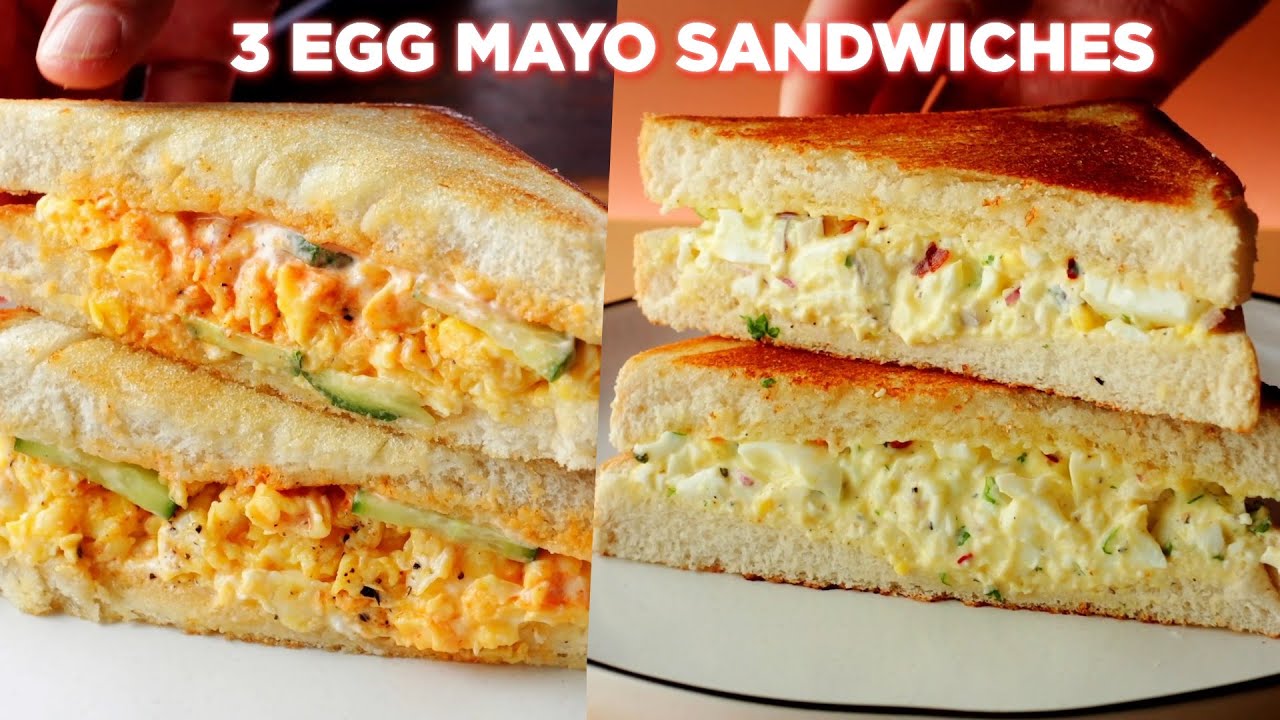The image is a composite of two pictures aligned side by side to form one larger image. At the top, in bold white letters with an orange stroke, the text reads "Three Egg Mayo Sandwiches." On the left side, there is a stack of two diagonally cut egg mayo sandwiches with toasted white bread. These sandwiches display a yellow egg mixture, featuring bits of cucumber and mayo. The background includes a visible hand, possibly grabbing the sandwich. On the right side, another stack of two diagonally cut sandwiches appears, also made of toasted white bread, but with a slightly more golden-brown crust. This right-side sandwich exhibits a more complex filling with a white-colored egg mix, red pepper pieces, black specks, and chopped greens, possibly green onions. The right image set is on a white circular plate, and similarly, a portion of a hand is visible in the background. Both sides show the sandwiches arranged and prepared with attention to detail, emphasizing the variety in toast level and sandwich fillings.